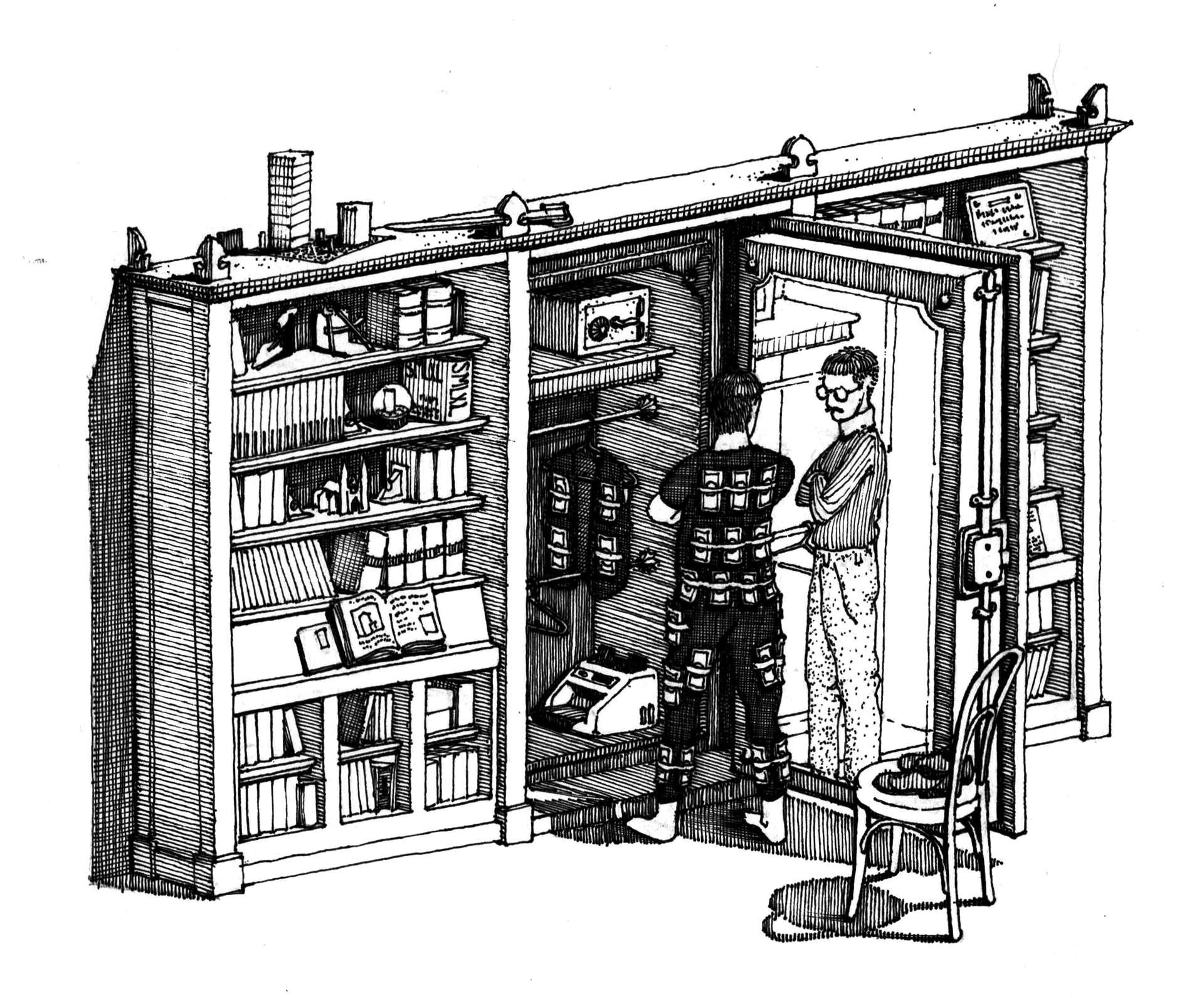In this intricately detailed black and white pen drawing that resembles a panel straight out of a Sunday newspaper cartoon, we are presented with a surreal and somewhat humorous scene. The setting appears to be a room featuring various objects, including a chair in the bottom right corner, an open door resembling a closet or a safe situated against a built-in bookshelf filled with books. 

At the center of the illustration stands a single man gazing into a mirror. Interestingly, while the actual man is bizarrely covered in what looks like mousetraps or possibly another object such as bombs, his reflection in the mirror appears completely normal. This juxtaposition highlights a peculiar contrast between reality and reflection. The real man’s attire seems unconventional—potentially pajamas—while the reflection showcases a typical outfit, including a black and white striped shirt and pants.

Additionally, small, indecipherable text can be found in the upper right section of the image, adding to the cartoonish and enigmatic atmosphere of the overall scene.